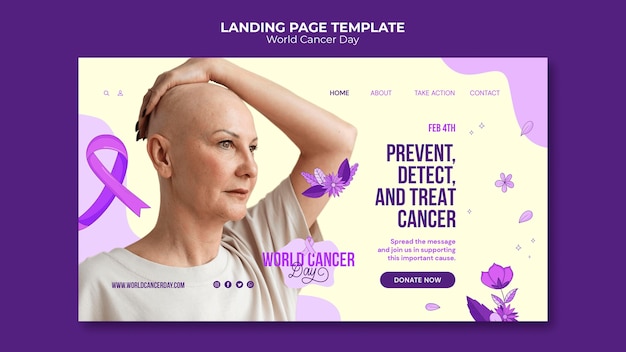The advertisement is a visually compelling purple-themed screenshot, resembling a postcard, designed to promote World Cancer Day. The primary background is a deep purple rectangle featuring bold white text that reads "Landing Page Template" at the top, followed by "World Cancer Day." Central to the image is a picture set against an off-white background adorned with subtle purple graphics, including a symbolic purple ribbon.

In the image, a woman in a beige top, with a bald head, signifying a cancer patient or survivor, gazes contemplatively to the side. She rests one arm on her head, with her palm touching her scalp. Below her image, "World Cancer Day" is reiterated to emphasize the theme of the advertisement.

Additional design elements include a navigation bar with links labeled Home, About, Take Action, and Contact. Under the main heading, it states "February 4th" to indicate the date of World Cancer Day, followed by the call to action: "Prevent, Detect, and Treat Cancer."

Decorative graphics such as small purple hearts and a purple flower enhance the aesthetic appeal. Beneath the heading "Spread the Message," a prominently placed "Donate Now" button encourages viewers to contribute to the cause. Social media icons and the website URL are also provided for further engagement.